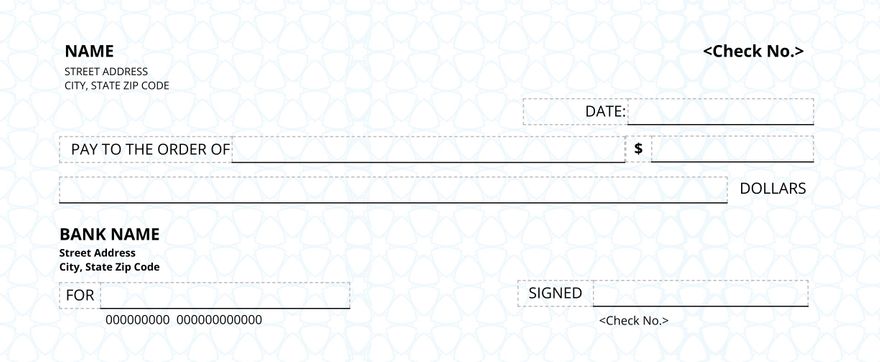This image depicts a blank check, characterized by its minimalist design and predominantly white background with subtle gray or light blue circular patterns. The check includes standard fields such as the name, street address, city, state, and zip code, which appear on the top left. On the top right, there is a space for the check number, followed by the date line. Below is the "Pay to the Order of" line, where the recipient's name is written, and adjacent to this is the amount box for inserting the monetary value in numbers. Further down, there is a line to write out the amount in words, designated with "Dollars." On the bottom left of the check, spaces are available for the bank name, street address, city, state, and zip code, and a line labeled "For" to denote the reason for the check. Finally, the space for the signature and an additional check number line are also present. Despite its essential features, the check maintains an unembellished, utilitarian appearance, making it clear that it is an outline ready to be filled in.